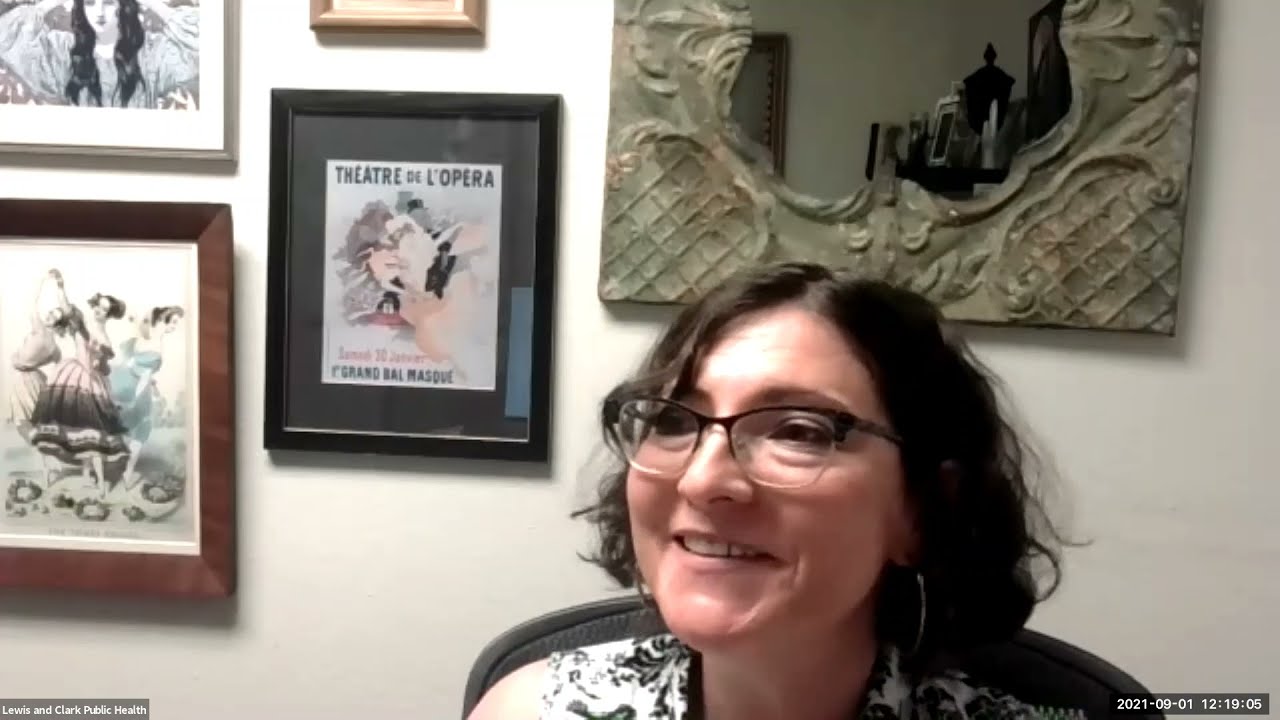In this screen capture from a video call, a woman in her mid-40s with wavy, dark brown, shoulder-length hair is smiling and possibly speaking. She is wearing horn-rimmed glasses with black frames on top and clear frames on the bottom. The woman, who is white, is seated in a gray chair and is dressed in a white shirt adorned with black floral patterns. Behind her, a white wall features four pieces of French-looking artwork, likely old play posters or theater art, with one partially cut out from the frame. To the right of the woman, a mirror with a clay-like frame edge captures a curved reflection of a background stand holding additional pictures and knickknacks. In the bottom left corner of the image, text reads "Lewis and Clark Public Health," while the bottom right corner displays a date and time stamp: "2021-09-01 12-19-05."